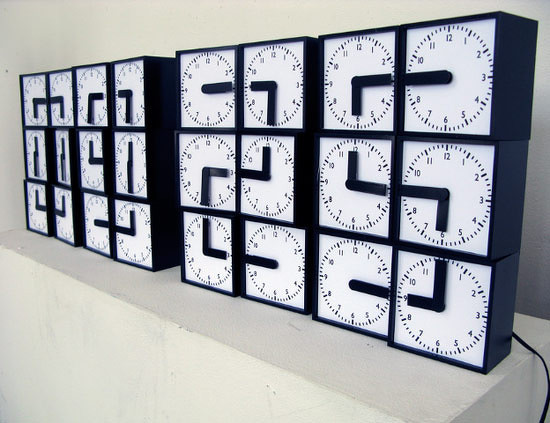The image depicts a slightly wider-than-tall, rectangular scene featuring 24 analog clocks, organized into four upright blue rectangular boxes, each containing six clocks arranged in a 2x3 grid. The arrangement of clocks forms a pattern resembling an LCD display, collectively displaying the numbers 0, 9, 2, and 5 from left to right. Each clock is white-faced with blue numerals and hands, while the background and supporting surface are white. A single black cord extends from behind the rightmost box, trailing off the bottom edge of the image. The clocks face the 10 o'clock position, creating a visual descent into the distance.